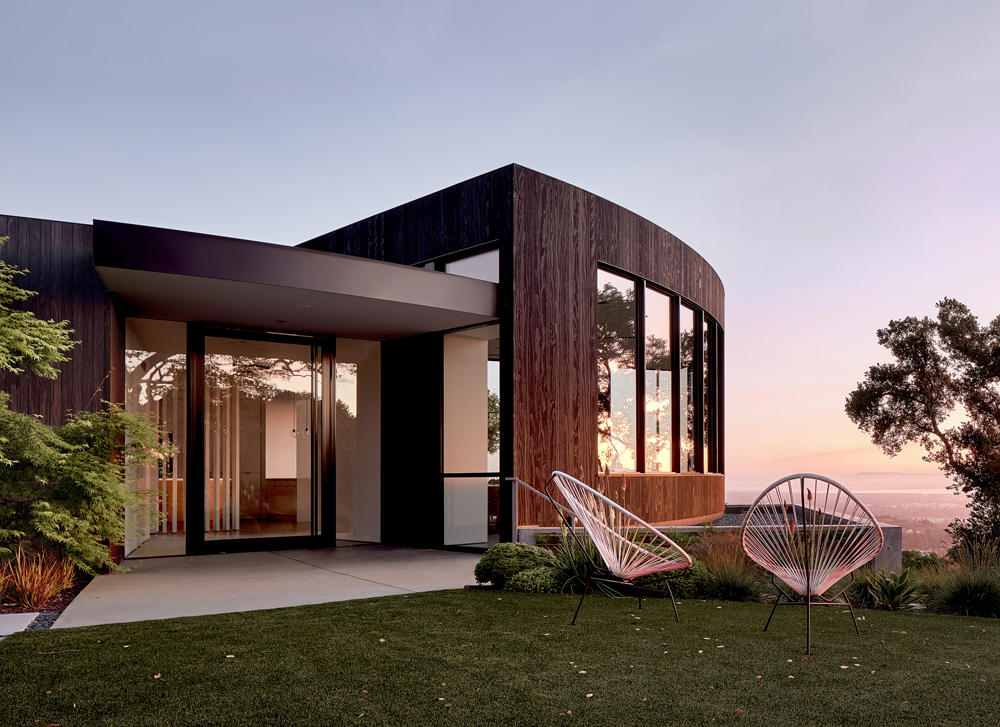This image shows a uniquely designed, contemporary house perched on a hillside, possibly overlooking a coastal city, with views of the ocean to the right. The house is strikingly modern with a flat roof and a distinctive blend of materials, featuring dark brown wood paneling, abundant glass windows, and possibly brushed metal elements. Its design includes a prominent curved, circular section on the right side, while the front has a large, floor-to-ceiling glass door trimmed in dark brown and covered by a small awning.

The landscape surrounding the house is well-maintained, with lush green grass, trees, and shrubs. The exterior includes a clean, white patio area and a concrete walkway. In the foreground, there are two modern, tulip-shaped metal chairs with circular frames, arranged to face the ocean, enhancing the serene, picturesque setting. The sky above is clear with shades of blue and pink, suggesting the photo was taken during twilight or sunset. Reflections of the trees and the softly lit horizon can be seen in the house's numerous windows, adding to the tranquil and luxurious atmosphere of this architecturally impressive home.